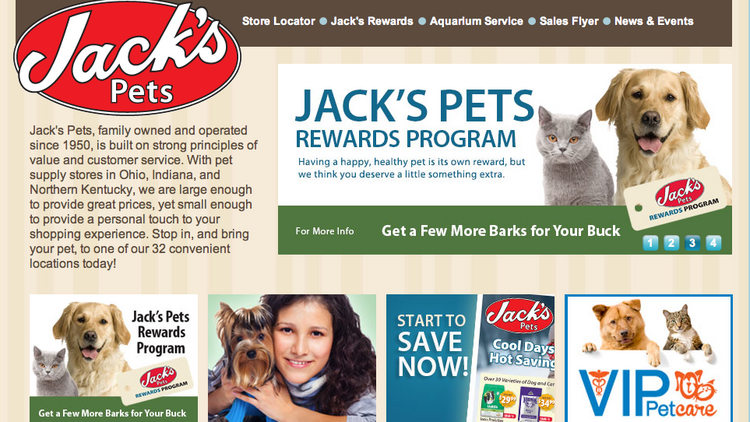The image captures a detailed screenshot of the Jax Pets website. At the top of the page is a brown border, with a red oval logo prominently displayed in the left corner. The logo features the word "Jax Pets" in white, with "Jax" being notably larger and occupying most of the oval. To the right of the logo, there are navigation options labeled: Store Locator, Jax Rewards, Aquarium Service, Sales Flyer, and News Events, each separated by blue circles.

Below the Jax Pets logo, there is introductory text that reads: "Jax Pets, family owned and operated since 1950, is built on strong principles of value and customer service with pet supply stores in Ohio, Indiana, and Northern Kentucky. We are large enough to provide great prices, yet small enough to provide a personal touch to your shopping experience. Stop in and bring your pet to one of our 32 convenient locations today."

On the right side, a rectangular banner advertises the "Jax Pets Rewards Program" and features an image of a gray cat and a golden retriever. Below this banner, a green border contains the text, "Get a few more barks for your buck."

At the bottom of the screen, four square images are displayed. The first square repeats the image of the gray cat and golden retriever and highlights the "Jax Pets Rewards Program." The second square shows a black-haired woman holding a small brown dog. Next to this, the third square contains an advertisement promoting the store with the text "Start to save now." The fourth and final square depicts a brown dog and a gray and white cat, with the text "VIP Pet Care."